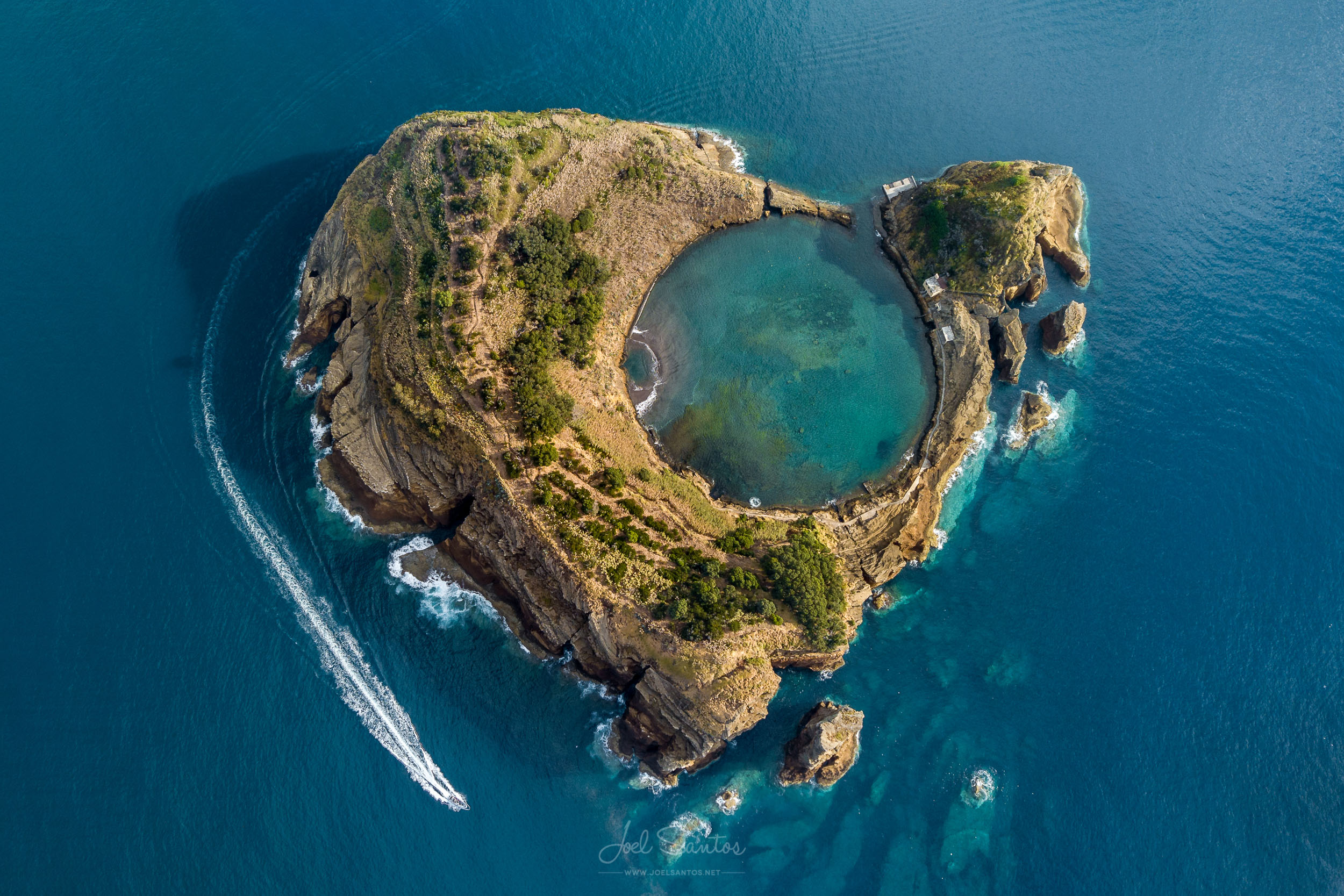The photograph, an aerial view taken on a sunny day, showcases a unique, heart-shaped island set amidst a vast expanse of dark blue ocean. The island, located on the left side of the image, is dominated by a tall, rocky mountain that gradually slopes down into a near-perfect circular lagoon connected to the surrounding ocean. Scattered trees adorn the island's terrain, enhancing its natural beauty. On the lower left side of the image, a speedboat leaves a white streak in the water, curving around the upper left corner of the island. A few rocky outcroppings can also be seen near the island. Additionally, the image features a watermark at the bottom reading "Joel Santos" along with a website name.